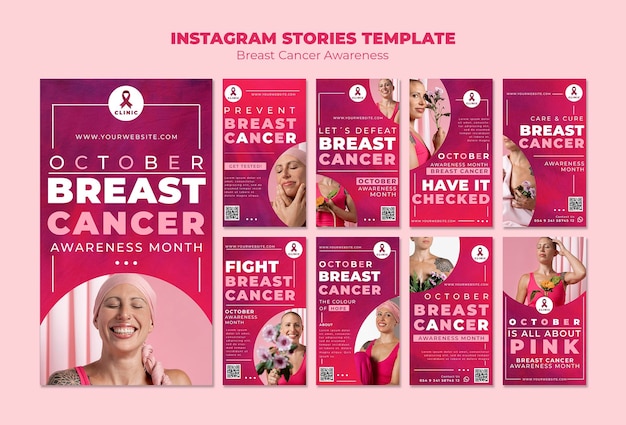This image showcases a set of Instagram Stories templates designed specifically for Breast Cancer Awareness Month. The overall background is a symbolic pink, reinforcing the cause's identifiable color. Dominating the center is a large, vertically oriented template adorned with a gradient transitioning from a rich maroon at the top to a pale red at the bottom. Within this template, a woman wearing a headscarf smiles broadly, her image framed by a half-circle cutout. The template is bordered by a delicate white line featuring the iconic cancer ribbon subtly integrated into the design. At the bottom, there is a placeholder for a website URL, along with the text "October Breast Cancer Awareness Month" displayed in an elegant mix of white and pink lettering.

Flanking this main template are eight smaller examples, each showcasing different configurations of the maroon-to-red gradient background and similar Breast Cancer Awareness themes. Each of these smaller templates also includes an image of a woman within a semicircular cutout, maintaining visual continuity across the set. These versatile templates provide a cohesive and visually appealing series of options for raising awareness and support during Breast Cancer Awareness Month on Instagram.